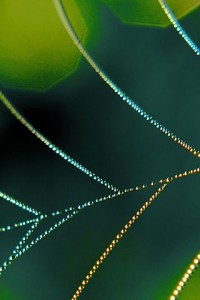This image captures an ultra close-up of a delicate spider web adorned with morning dew, creating an array of sparkling droplets. The background features a blend of dark and light green foliage, forming shapes that almost appear geometric due to the extreme zoom, making it challenging to distinguish individual elements. The spider web's intricate strands glisten with silver hues, possibly reflecting a spectrum of colors due to the light shining upon them. The scenery suggests a natural setting, enhancing the ethereal beauty of the web suspended in mid-air. The ambiguity of whether the threads belong to a spider web or the veins of a leaf adds an intriguing layer of mystery to the image. The composition’s color palette includes shades of green, black, silver, and hints of bronze, offering a visually captivating snapshot that blurs the lines between reality and abstraction.